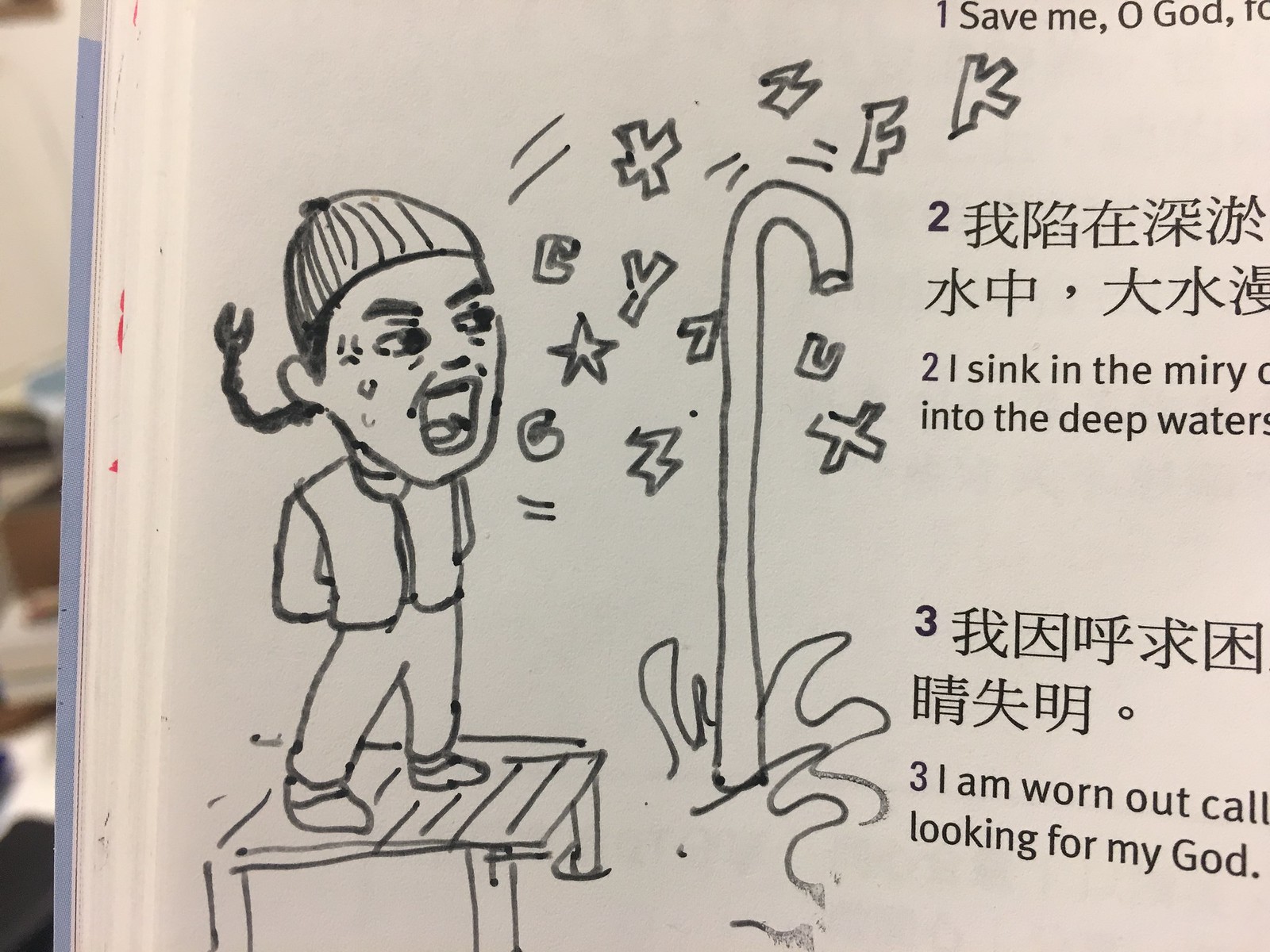This detailed black and white drawing, created with markers, depicts a woman standing on a wooden table. She appears to be shouting, as evidenced by her wide-open mouth and a stream of various letters, including "E-X-Y-7-C," "Z-F-K-U-X," and symbols like stars and zigzags emerging from it. The woman has thick eyebrows and is slightly in profile, with her eyes looking to the right. Her hair is styled in a braid with an upward bend, resembling a claw, and she's wearing a beanie hat, a vest or jacket, and pants. Behind her, a large hook-shaped object resembling a faucet is drawn, with what looks like moving water at the bottom. The drawing is on a pastel blue and white book or board, and there are visible inscriptions in a foreign language, along with the phrases "Save me, O God, F-O" and "I sink into the deep waters. I am worn out, call looking for my God." The scene is framed by a white wooden edge on the left side.